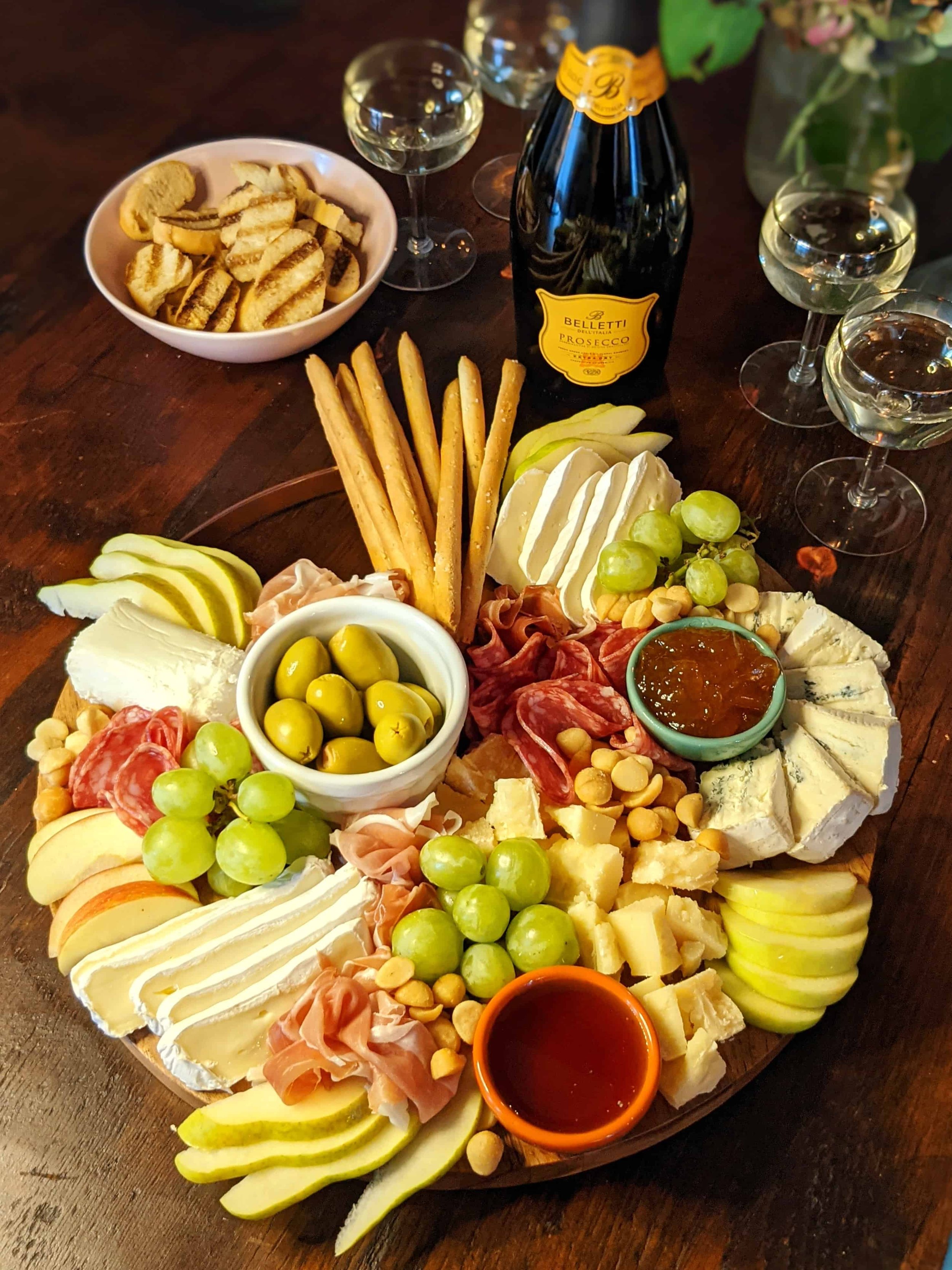This photograph captures a delectable charcuterie spread presented on a dark wooden table. Central to the scene is a rounded platter brimming with a variety of cheeses, charcuterie meats such as salami, green grapes, apple slices, nuts, and breadsticks. Nestled among these are several small bowls: a white bowl holding light green olives, a green bowl containing red pepper jelly, and another bowl with a different kind of sauce. On the top left of the platter, there is a brown-colored bowl filled with long, brown pretzel-like breadsticks. Adjacent to them, some slices of a white and yellow food item are visible. An orange container with a red liquid also features towards the bottom right of the spread.

Complementing the charcuterie board is a bottle of Valetti Prosecco, positioned behind the platter. The bottle features a distinguishable dark black and yellow label. Surrounding the bottle are four glasses that appear to be filled with either Prosecco or water, given their light, transparent appearance. Additionally, a pink bowl, seemingly filled with crispy bread pieces with slight burn marks, is placed in the upper left corner of the image.

In the upper part of the photo, a partial view of a vase, likely containing flowers, adds a subtle aesthetic touch, even though the flowers themselves are cut off from the frame. The entire setup exudes a tasteful and inviting ambiance, making it a perfect feature for a cooking blog or website.